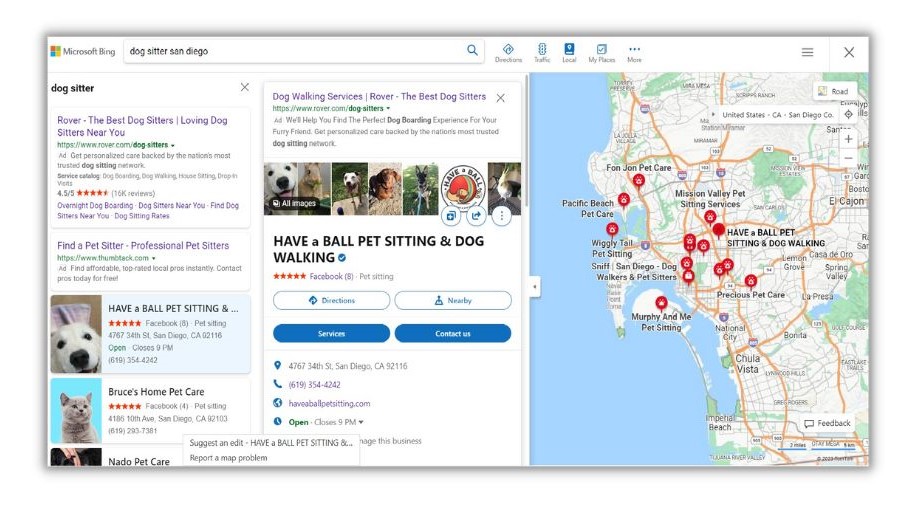The image is a landscape-oriented screenshot of a search result page from Microsoft Bing. The rectangular screenshot is framed by a gray shadow-like border and is approximately twice as long as it is tall. In the upper left-hand corner, a Microsoft Bing icon featuring the Microsoft flag is visible, followed by a white search box containing the query "dog sitter San Diego" in black font and a search icon.

Below the search bar, there are several icons. While some are indistinguishable, one notable icon says "directions," accompanied by three additional option icons and a "more" button, with a hamburger menu situated to the left.

The left side of the screenshot features a vertical white column listing search results. The first result is a link to the website Rover, displayed in blue text, with a green description link beneath it and a rating of 4.5 out of 5 stars. Below that, another result prompts users to "find a professional sitter," listing several entries with additional details beneath each.

To the right of this column, a search result is highlighted, leading to a web page named "Happy Ball Pet Sitting and Dog Walking." This section includes images of dogs along with links to directions, nearby services, and a "Contact Us" option, complete with the address and phone number of the service.

On the far right of the screenshot, a map is displayed, showing different pet sitting services marked by pinpoints, providing a geographic context for the search results.